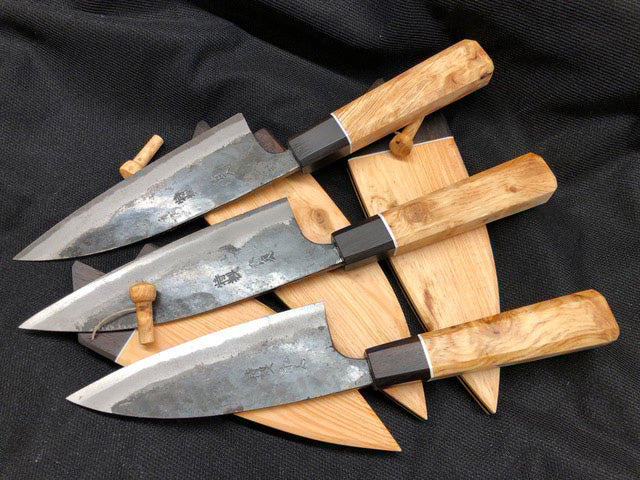In this image, a neatly arranged set of three identical knives is displayed, each oriented with the blade pointing towards the bottom left corner and the handles towards the top right. The handles are crafted from light brown wood, exuding a warm and natural aesthetic. The blades gleam with a sharp, steel-like brilliance, and intricate foreign characters, which seem to be Japanese or Chinese, are etched along their expanse. Positioned beneath each knife are their respective sheaths, matching the light wooden hue of the handles. The entire setup rests upon a textured black cloth, providing a striking contrast that accentuates the elegance of the knives.